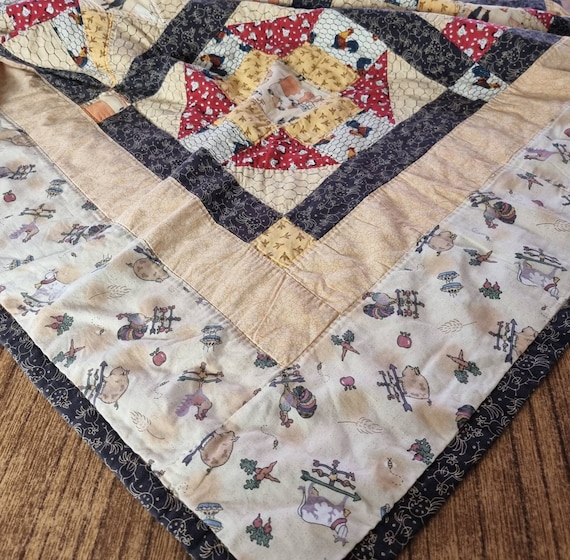This image features a multi-colored quilt laid out on a brown, wood-paneled floor. The quilt, covering most of the picture, is composed of several layers of intricate patterns. Around the edge, a dark grayish-black border adorned with designs resembling small insects or ladybugs encases the quilt. Within this border, the first sequence of patterns includes images of farm animals such as pigs, cows, and chickens, as well as fruits like apples and food items like pies. Various hues and nude colors dominate the quilt's layers. Beyond the farm-themed layer, a beige ribbon is followed by another dark border. Towards the center, geometric patterns emerge, featuring triangles and small squares, with a recurring motif of chickens set against alternating black and white backgrounds. The central design is a complex arrangement of red and white geometric shapes, creating a visually engaging composition.